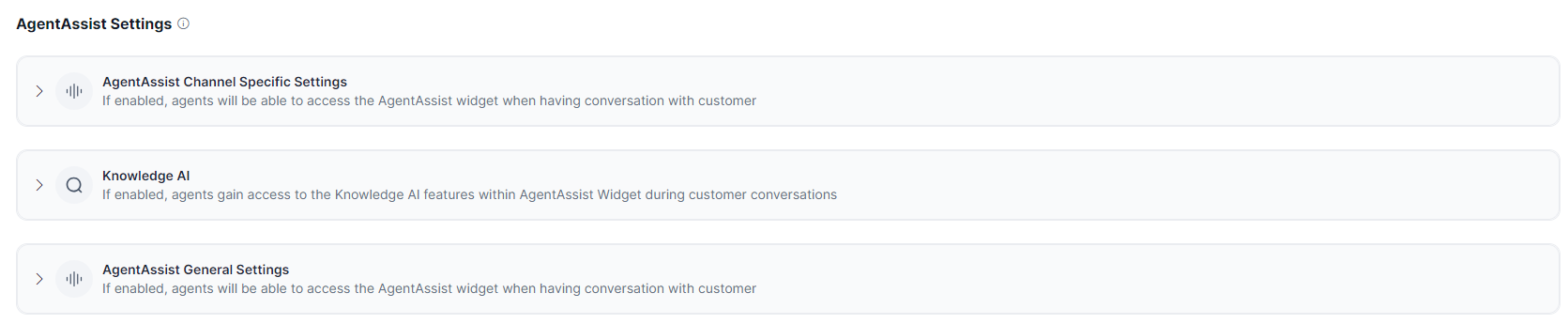This detailed image displays a structured layout with text and settings related to an agent assist system. The background is white, providing a clear contrast to the bolded black text positioned in the upper left corner that reads "Agent Assist Settings." 

Directly below this, there is a pale gray box labeled "Agent Assist Channel Specific Settings." Within this box, it describes that if the setting is enabled, agents will have access to the agent assist widget while conversing with customers.

The next highlighted gray box is titled "Knowledge AI." This section explains that enabling this setting allows agents to utilize Knowledge AI features within the agent assist widget during customer interactions. To the left of this box, there is a small magnifying glass icon.

The final element is a gray box beneath "Knowledge AI," labeled "Agent Assist General Settings." Similar to the previous sections, this box indicates that if the setting is enabled, agents can access the agent assist widget during conversations with customers.